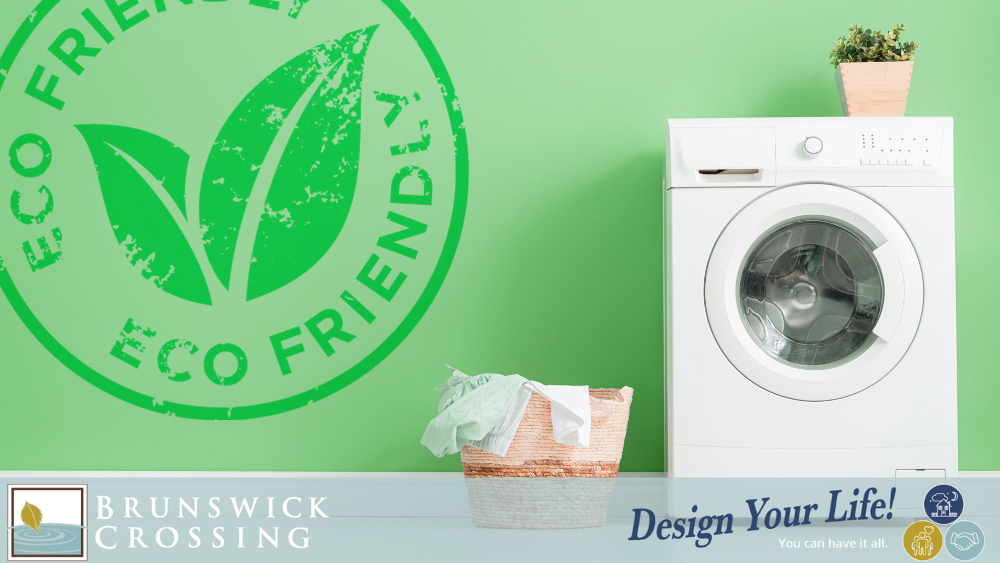The advertisement image features a vibrant lime green background, with an eco-friendly icon prominently displayed in the upper left corner. The icon consists of a light green circle encasing two green leaves with a white stem. Centered in the image is a wicker laundry basket overflowing with white clothes. To its right stands a modern white front-loading washing machine adorned with a potted plant in a natural wooden base on top, giving it a stylish, eco-conscious vibe.

At the bottom of the image, a grey bar stretches across with the branding elements. On the left side of this bar is a logo depicting a square with a leaf and circular water motif. Next to this, white text on a blue background reads "Brunswick Crossing." Further to the right, bold text states "Design Your Life," accompanied by the tagline "You can have it all." Additionally, three circular icons align under this text, representing different concepts with imagery like a house, family stick figures, and leaf-shaped hands, emphasizing a comprehensive lifestyle message.